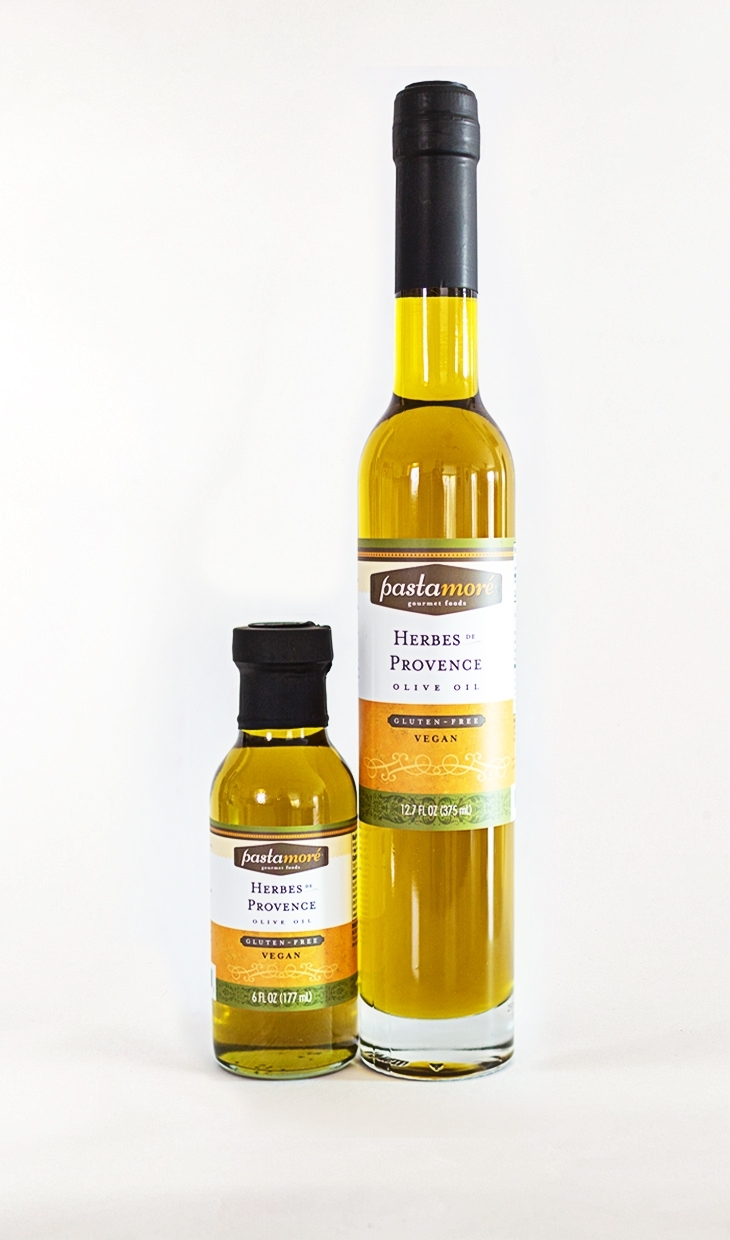The image features two olive oil bottles from Pastamore Gourmet Foods, styled as Herbs de Provence Olive Oil. The bottles are set against a plain, light grey background and are standing side by side. The bottle on the left is a shorter, sample-sized bottle containing 6 fluid ounces of olive oil, while the bottle on the right is a taller one with a capacity of 12.7 fluid ounces and resembles the height and neck shape of a wine bottle. The olive oil inside both bottles exhibits a greenish-yellow hue. Both bottles feature identical labels with a series of stripes—green, dark green, orange, and dark orange—and include the text "Herbs de Provence, Olive Oil, Gluten-Free, Vegan." Each bottle is fitted with a black cap with a tapered seal around it, adding an elegant touch to their appearance.